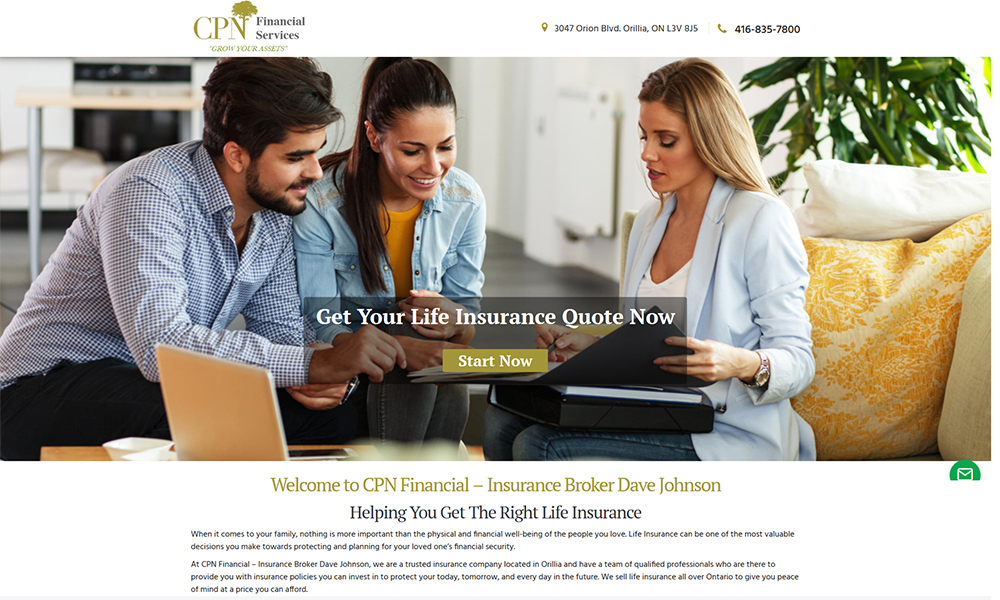The image appears to be a screenshot of a website, featuring a detailed header and main content area. The header is indented from the top and includes a logo on the left with the text "CPN Financial Services." Off-center to the right are the details "3047 Onion Boulevard, Villa Ontario, L3V Beach JS," although the print is small and hard to decipher. Next to this address is a phone icon followed by the number "416-835-7800."

Dominating the main screen is a photograph showcasing a man and a woman seated side-by-side, intently looking at a portfolio being shown to them by another woman. Overlaying this image is the text "Get your life insurance quote now," accompanied by a clickable "Start Now" button. Below this overlay, there's text that reads: "Welcome to CPN Financial Insurance broker Dave Johnson helping you get the right life insurance." Beneath this welcome message are a couple of paragraphs in small font, which are illegible.

The man in the image is dressed in a blue plaid check shirt and has dark hair and a beard. The woman next to him, with dark hair as well, is wearing a light blue button-up sweater over an orange shirt. The woman presenting the portfolio is attired in jeans, a business suit jacket, and a white t-shirt, and she sports a watch on her left wrist. She is seated on a couch, while the couple appears to be sitting on a footstool. A laptop is visible on a coffee table in front of them, adding to the office-like setting of the scene.